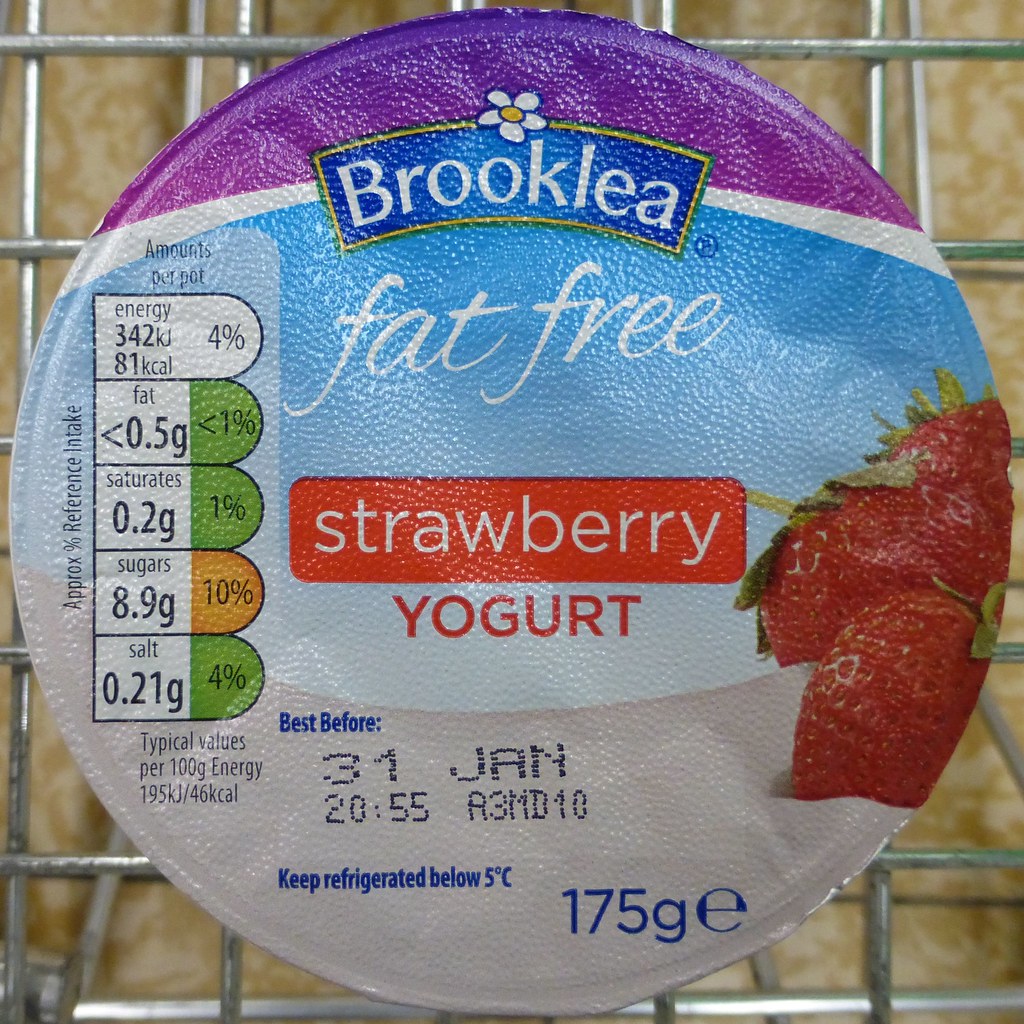The image showcases a detailed, overhead view of a Brook-Lea fat-free strawberry yogurt container lid set against a backdrop of metal wiring from what appears to be a shopping cart. The lid is centered in the picture and displays a vibrant collage of colors including light blue, dark blue, yellow, red, purple, and green. At the top of the lid, there is a blue banner outlined in yellow, featuring a white daisy and the text "Brook-Lea." A purple line, followed by a white stripe, separates this from the sky-blue background.

Further down, in bold white letters, the words "fat-free" stand out. A red banner with white text beneath this denotes "strawberry," followed by another red section that reads "yogurt." To the right, images of fresh strawberries add a touch of realism and color contrast to the design. To the left, the nutritional profile is elaborately listed, featuring energy content (342 kJ, 81 kcal, 4%), fat (0.5 grams, under 1%), saturates (0.2 grams, 1%), sugars (8.9 grams, 10%), and salt (0.21 grams, 4%). This is accompanied by a vertical text indicating "Approximate Percentage Reference Intake" in black.

At the bottom, a blue text states "Best Before," followed by a black print with the expiry date "31 January 2055 A3MD10." Additional instructions appear in blue, instructing to "Keep Refrigerated below 5 degrees Celsius," along with the weight "175 grams."

Gray metal wiring frames the yogurt lid, suggesting the container is placed in a shopping cart. The collective details and vibrant colors of the image create a clear and informative visual representation of the yogurt container’s top label.